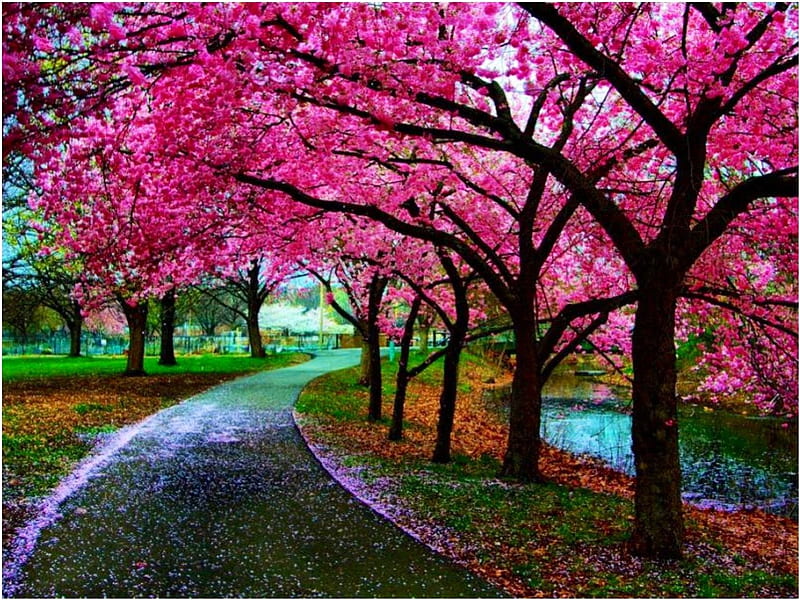This photograph, possibly enhanced for vividness, depicts a serene and colorful park scene with a curving asphalt pathway that meanders through an enchanting canopy of blossoming trees. These trees, likely cherry blossoms, exhibit brilliant fuchsia pink flowers, creating a mesmerizing tunnel that arches over the path. The ground is sprinkled with a pretty dusting of these pink petals, adding to the enchanting effect. 

The park features diverse foliage; vibrant green grass competes with fallen orange, brown, and yellow leaves, enhancing the tapestry of colors. To the right of the path, a tranquil pond mirrors the sky in blue and green hues, its surface dotted with petals and leaves. Dark tree trunks and sprawling branches frame the vivid floral display, amplifying the contrast and highlighting the blossoms' beauty.

The scene is completed with glimpses of green lawns and sparse buildings in the blurred background, suggesting a transition from the natural enclave closer to civilization. The sky peeks through the dense foliage, indicating a bright, cloud-spotted day, further elevating the colors in this beautifully detailed park scene.